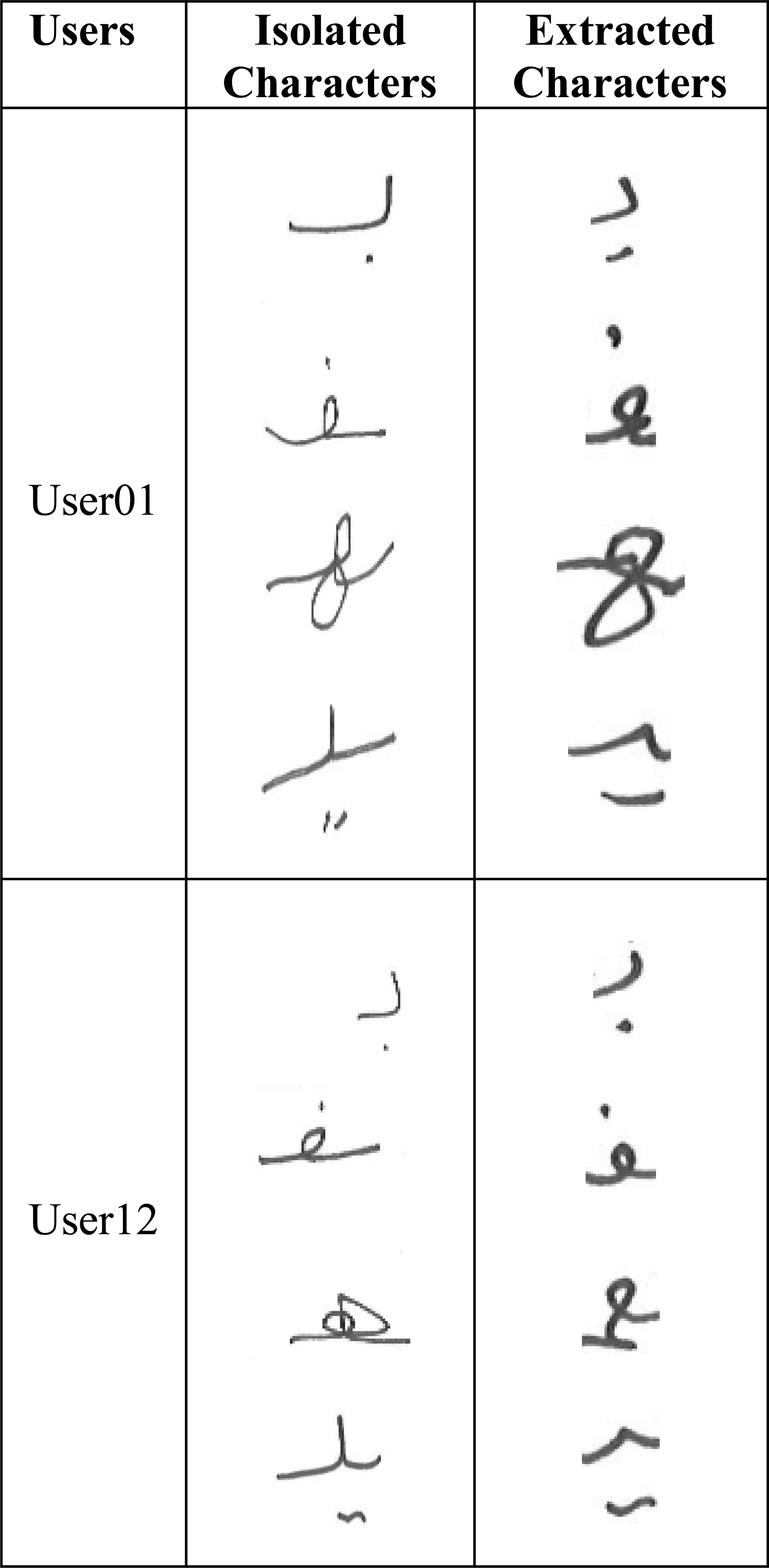The image features a chart on a white background, divided into three main columns and two rows. At the top of the chart, there are three rectangular boxes with bold, dark black text. The first and narrower box is labeled "Users," the middle box is labeled "Isolated Characters," and the box on the right is labeled "Extracted Characters." Under the "Users" column, two rows are labeled "User01" and "User12." The "Isolated Characters" and "Extracted Characters" columns contain handwritten symbols that do not resemble standard English letters, suggesting they could be from another language or shorthand. Notably, under "User01," there is an 'F' in cursive. Another character looks like an 'E' with a dot over it, while its counterpart in the "Extracted Characters" column appears more upright. The symbols in the "Extracted Characters" column are similar to those in the "Isolated Characters" column but are bolder. Under "User12," similar patterns are observed with slight variations, including symbols that resemble cursive letters and other unfamiliar marks.